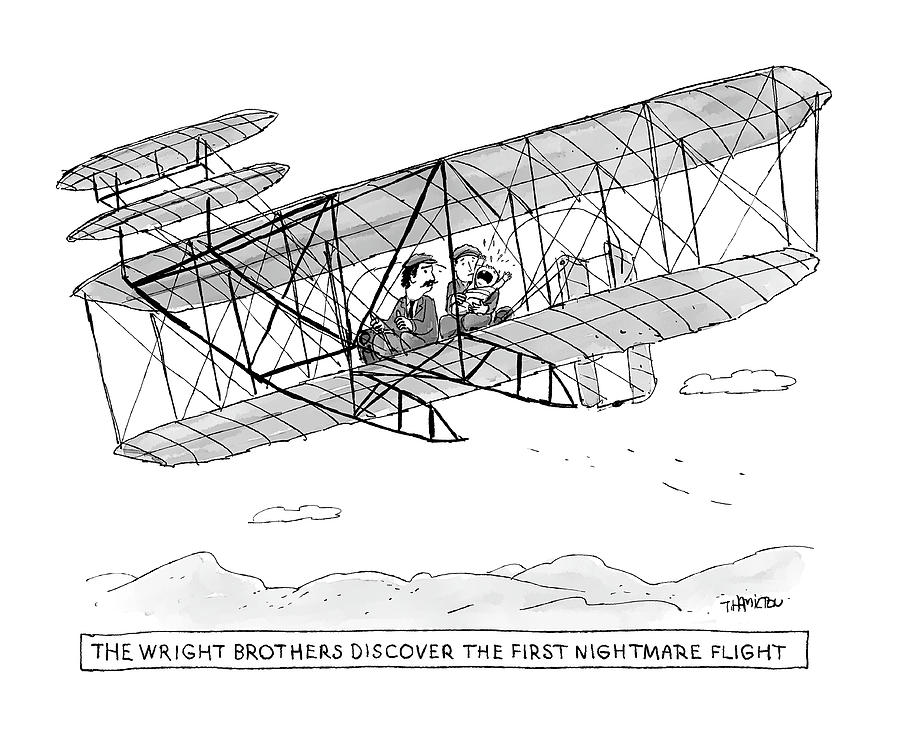This pencil sketch, resembling an old-school one-panel newspaper cartoon, humorously depicts the Wright Brothers' first flight with a comically nightmarish twist. Against a largely white background, a rudimentary depiction of their historical plane is finely detailed, featuring characteristic lattice work and thin wing panels. The Wright Brothers sit mid-plane, positioned on the wings, incongruously accompanied by a crying baby, which one of them holds as they both look helplessly at each other. This playful anachronism is underscored by the caption "The Wright Brothers discover the first nightmare flight" framed in black text. In the background, minimalistic clouds float above modestly illustrated mountain ranges, adding a touch of scenery. The image bears the signature "THAMICTOU," suggesting the artist's name.